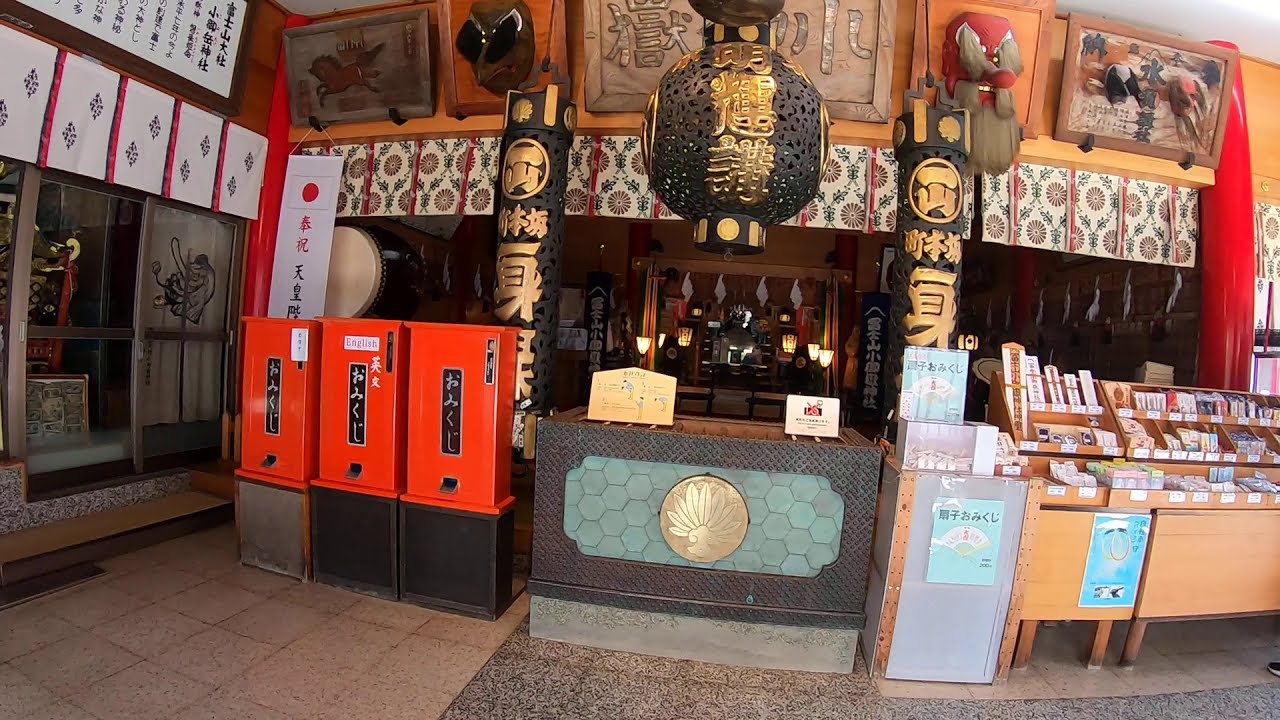This photograph captures a richly decorated Chinese shop, taken from its exterior which creates an impression of looking into an outdoor but semi-enclosed space. The shopfront is elegantly adorned, featuring a prominent circular black decorative item hanging from the roof, inscribed with golden Chinese characters. Two sturdy pillars stand in the garden-like outer structure, also bearing Chinese characters in gold. 

The floor outside the shop consists of an intricate pattern of square tiles in shades of brown and grey, transitioning to a mottled dark brown towards one side. At the entrance, a sliding glass door is framed by white banners with red trim and diamond shapes, topped with a large wooden scroll showcasing Asian script.

Noteworthy, the shop interior is vibrant with lights and lamps visible from outside. A variety of items are displayed: three red vending machines with Japanese writing, and a countertop adorned with a gold medallion and blue tiles, suggesting a place where customers are served. Above the shop, different pictures and framed photographs, including one of a horse, along with unique masks resembling a bird and a Tengu monster, are displayed. Complementing the rich decor are black metal works, including a large black metal ball and two elongated cylinders, all featuring golden inscriptions.

Stools positioned outside the shop carry various goods, and an incense stand is noticeable on the right. Overall, the detailed setup of the shop creates a culturally immersive experience through its intricate design elements and curated displays.